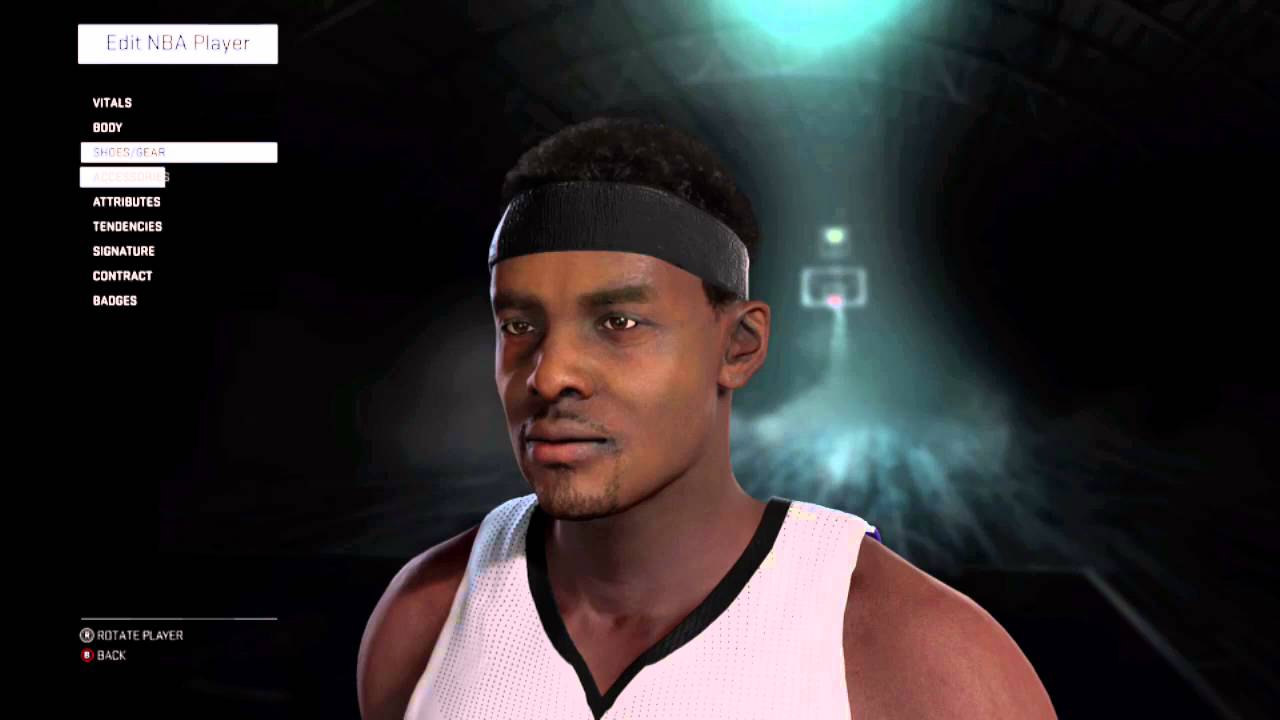In this image, you see a rectangular frame oriented from left to right, predominantly filled with black space. Positioned towards the left central area stands an African American man, whose gaze is directed as if he is looking to the left of the image. Behind him, bathed in a green light, you can make out the blurred silhouette of a basketball hoop, suggesting that the setting is a basketball court. The man is wearing a black headband and sports faint facial hair, including a subtle goatee. He is dressed in a white sleeveless top with a black neckline, resembling a waffle texture, and only the upper portion of his body is visible in the frame. 

On the left side of the image, starting at the top, is a white box containing the text "Edit NBA Player." Below this, additional text categories are listed: "Vitals," "Body," "Attributes," "Tendencies," "Signature," "Contract," and "Badges," indicating elements likely related to a player customization or statistics screen, possibly in a video game.